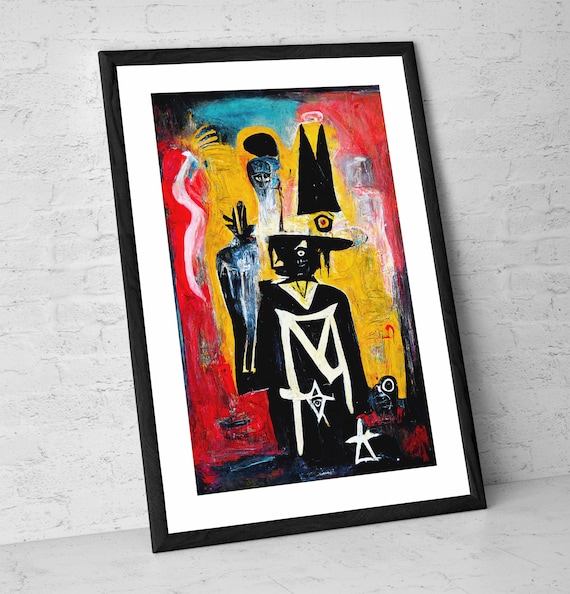In this photograph, a painting leans against a white brick wall. The painting, enclosed in a dark brown wooden frame, features a chaotic array of horror-themed elements and vivid colors, predominantly red, yellow, blue, and black. The central character is a sinister figure draped in a black robe adorned with white lines, raising a hand suggestively, possibly invoking religious or mystical symbolism. Around this figure, a host of eerie entities such as ghosts, goblins, and skeletons populate the scene, each rendered in bold, unsettling compositions. Notable details include a large-eyed bird head in the lower right-hand corner and a black shirt with a white diamond featuring an ominous eye at its center. A masked figure also emerges from the scene, adding to the macabre ambiance. The painting's abstract nature and its evocation of horror make it reminiscent of Halloween-themed artwork, replete with mystical evil eyes and bizarre creatures.